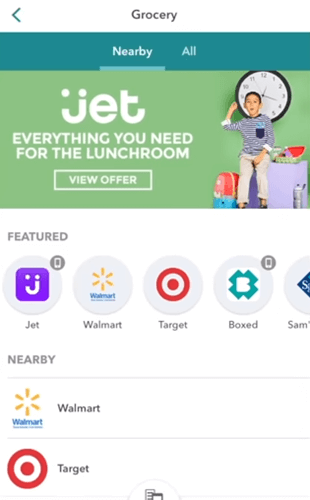The image appears to be a screenshot from a mobile phone. In the top left corner, there is a back arrow icon. Centered at the top, the word "Grocery" is displayed. Below this, on a dark greenish-blue background, there is a sorting option with "Nearby" selected instead of "All." 

Beneath this, a section with a green background features a banner for "JET," promoting "everything you need for the lunch room with a view," displayed next to a child wearing a blue shirt and tan pants, who stands in front of a clock and is surrounded by shopping bags.

Further down, on a white background, there is a list of featured stores displayed within circles. On the left, "Featured" is indicated, followed by a series of circular icons with store logos: 
- A purple square with a smiley face and the label "JET"
- The Walmart logo, featuring the sun icon and the word "Walmart"
- Target's red bullseye logo
- Boxed's logo, which seems like a sideways plus sign with a "B"

Below these featured stores, the "Nearby" section lists specific stores with similar presentation:
- "Walmart" with its icon on the left
- A line separator
- "Target" with its bullseye logo on the left